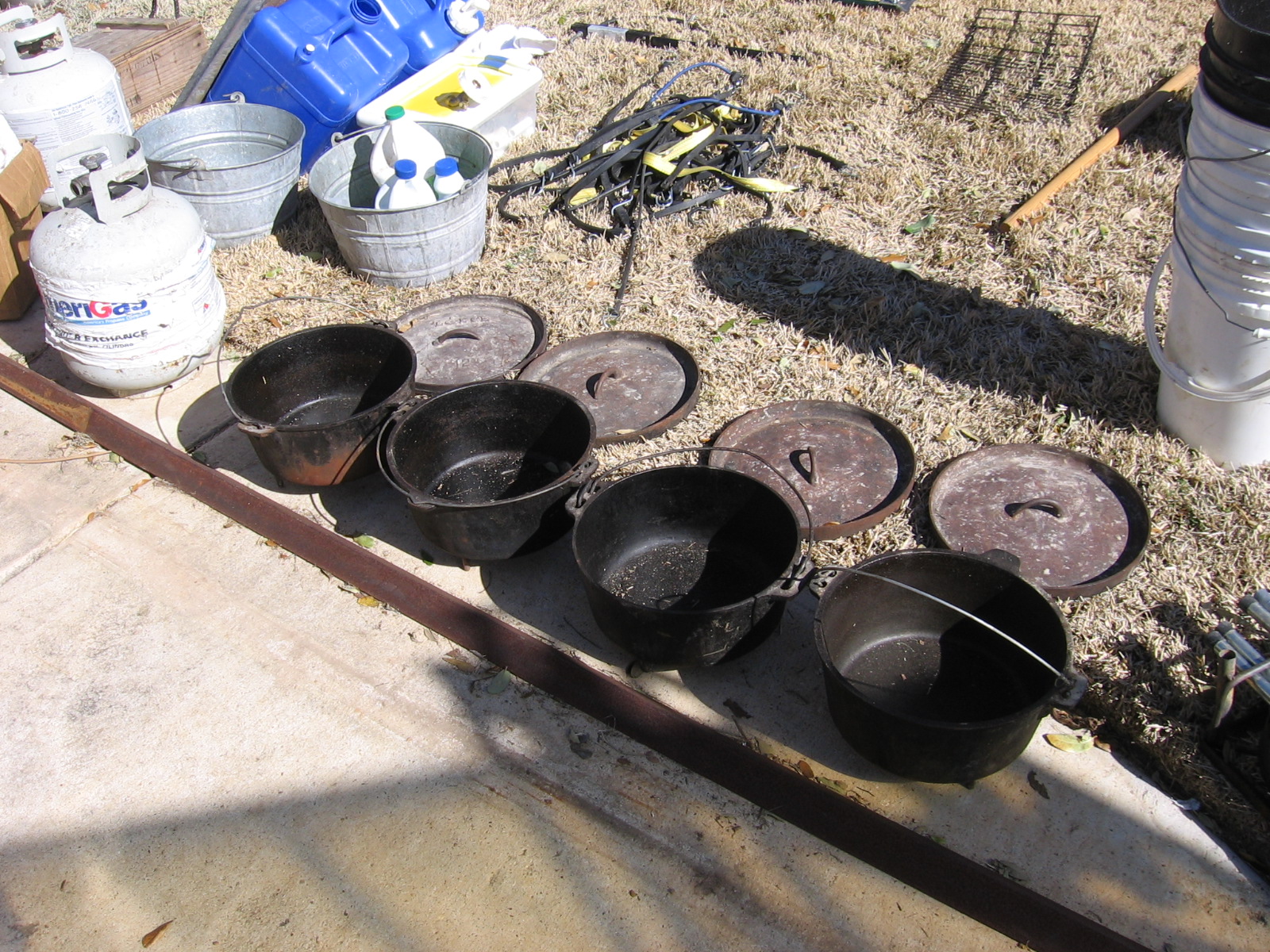This outdoor photograph, taken in bright sunlight, prominently features a concrete sidewalk that occupies the lower left-hand side to the middle of the image. Running parallel along the edge of the sidewalk are four old, well-seasoned cast iron pots, each with a thin wire handle. Their cast iron lids, which appear rusty, are set on the dried, light brown grass directly in front of each pot. To the upper right part of the image, on the grass, are various items: several white plastic buckets stacked in the far corner, a pair of large Amerigas propane tanks on the left—one closer, one farther back—and a couple of galvanized metal wash buckets, one of which contains three white bottles resembling bleach bottles with blue caps. Additionally, scattered around are random objects like black cords, an item that looks like a broom handle, and open blue water containers. Shadows of these objects indicate the bright, sunny conditions under which the photograph was taken.